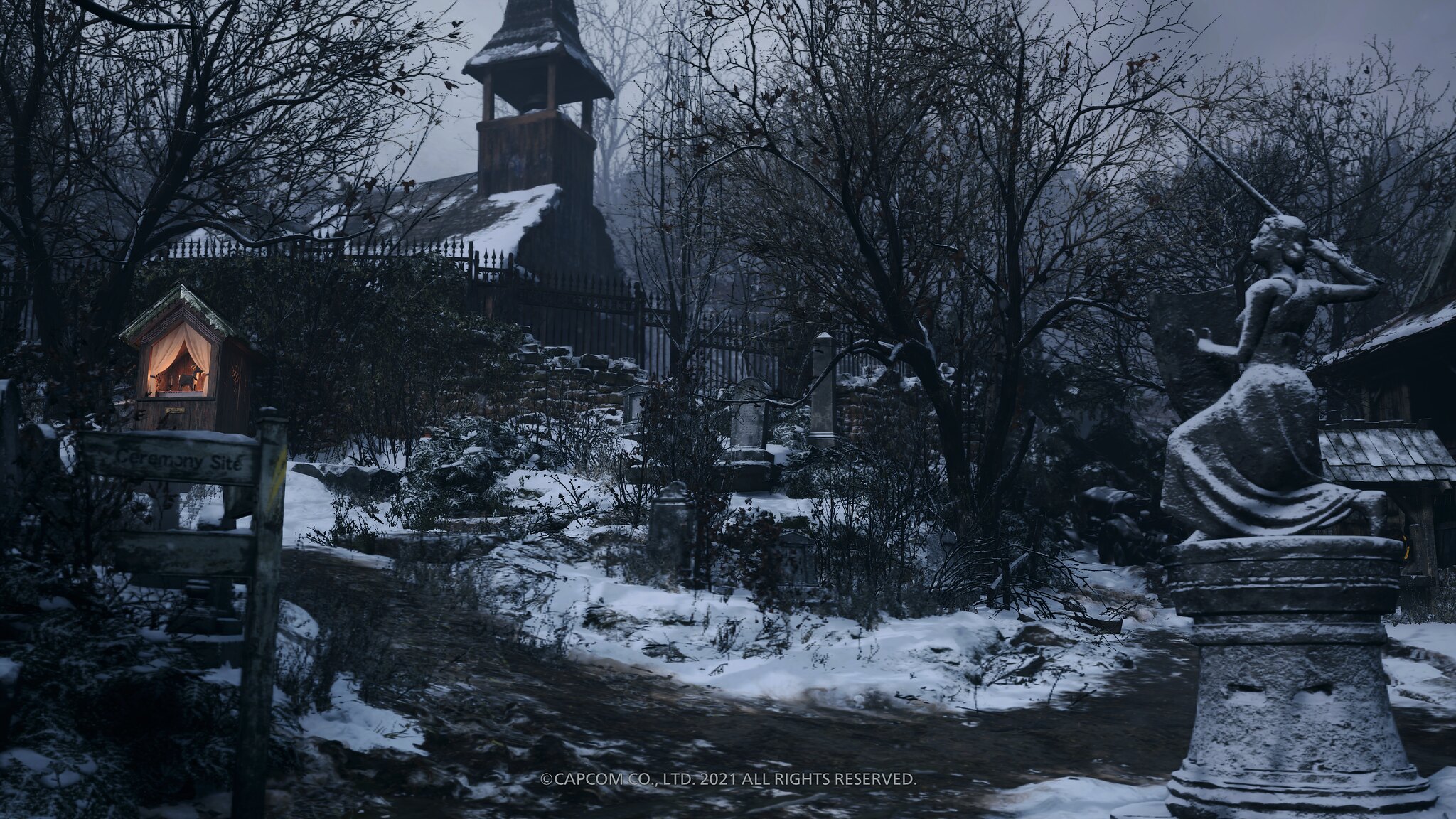The image appears to be a screenshot from a video game, bearing the copyright notice "© Capcom Co., Ltd. 2021 All Rights Reserved" at the bottom in white lettering. The scene is set in a cold, snowy environment, with a gray, overcast sky. Dominating the background is an old church building featuring what seems to be a bell tower. 

In the foreground, there’s a cemetery with numerous gray tombstones scattered on snow-covered ground, creating a somber atmosphere. To the right, there stands a detailed statue of a woman. She is depicted wearing a long robe, kneeling with her right knee on a cylindrical pedestal while her left leg is bent. The statue holds a spear in her right hand and a shield in her left hand. The area is surrounded by leafless, black trees and scrubby vegetation, heightening the desolate mood of the scene.

There are also other structures: a smaller house with a snow-covered roof and a spiked black fence, and a brown house with white curtains glowing with light from within. Additionally, a pole with signs, one reading "Ceremony Site," stands to the left, completing the eerie, abandoned atmosphere of this wintry tableau.